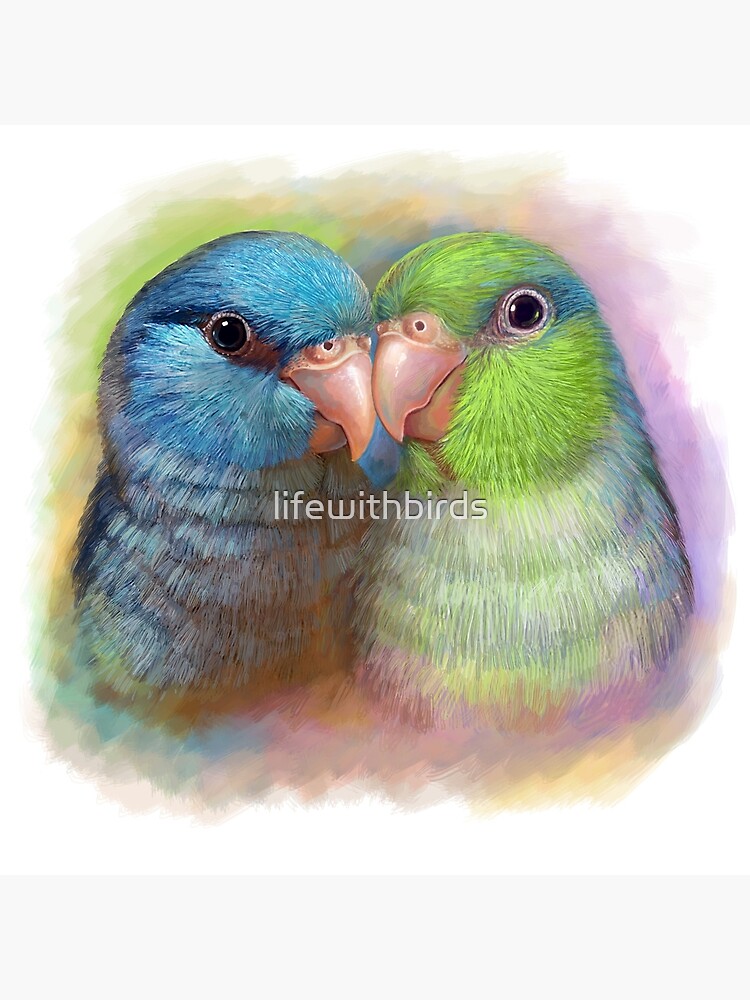The image is a detailed watercolor painting featuring two affectionate parakeets prominently displayed in the center. The parakeets, composed in soft and vibrant hues, appear to be nestling or gently touching beaks, evoking a sense of intimacy and tenderness. The bird on the left is primarily light blue with variations of darker blue throughout its feathers, transitioning to an off-white hue towards its lower body. Its beak is a light brown, and it has a single visible eye with a dark pupil encircled by white. The parakeet on the right contrasts with a predominantly light green plumage, streaked with shades of darker green and touches of blue, especially around its eye, which also has a black pupil bordered by white. This parakeet's beak matches the light brown of its companion's, and its body transitions to an off-white color near the neck. Below their beaks, the phrase "Life with Birds" is inscribed in an off-white color without any spaces between the words. The background is a harmonious blend of blurred watercolor blotches encompassing hues of green, purple, yellow, and orange, which frame the birds against a primary white backdrop, enhancing the painting's delicate and lovely composition.